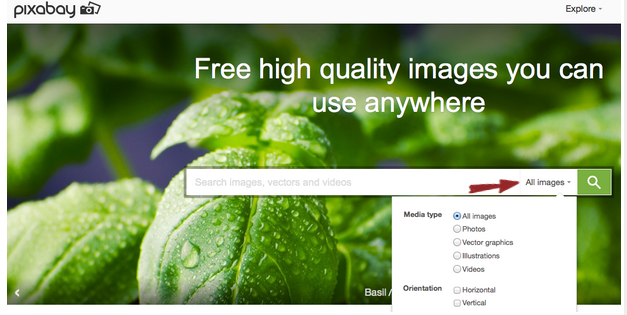The website features a detailed layout with a focus on image exploration. In the upper left corner, the website’s logo "Pixabay" is displayed, accompanied by a small black camera icon. On the upper right side, there's an "Explore" button in black text with a gray downward arrow beside it. 

The background showcases a muted image of vibrant green leaves, close-up, adorned with water droplets. Superimposed across this leafy backdrop is a white banner with the text "Search Images, Vectors, and Videos." Accompanying this text is a red arrow pointing to "All Images," next to a small green arrow pointing down. Moreover, there's a green box featuring a white search icon.

Below this banner, a user-generated pop-up appears labeled "Media Type" in black text. This section includes "All Images" with a blue filled circle next to it and a red arrow pointing towards it from the banner above. Below, categories such as "Photos," "Vector Graphics," "Illustrations," and "Videos" are listed but without colored circles. 

Additional sections labeled "Orientation" follow, with options for "Horizontal" and "Vertical," both of which remain unchecked. In the background, faint text emerges beneath the "Media Type" and "Orientation" labels, revealing the word "Basal," suggesting that the green leaves depicted belong to a basal plant.